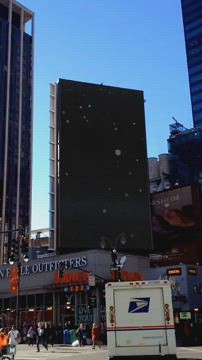In this daytime photograph of a bustling city street, the viewer's attention is immediately drawn to the front of an Outfitters store. Centered in the foreground is a USPS white truck with its back facing the camera, featuring the recognizable blue and white Eagle emblem prominently displayed on its closed rear door. The street is alive with activity as multiple pedestrians amble and interact, creating a lively urban atmosphere.

Adjacent to the scene, street crossing signals and traffic lights are clearly visible at the street corner, indicating organized mobility for vehicles and pedestrians alike. The cityscape is framed by taller buildings flanking the view on both the left and right sides, suggesting a vibrant downtown area. Dominating the center of the photo is a large, rectangular billboard adorned solely with a black and white star pattern, adding a unique visual element to the urban setting. The composition of the image captures the dynamic energy of city life framed by both functional and decorative urban fixtures.